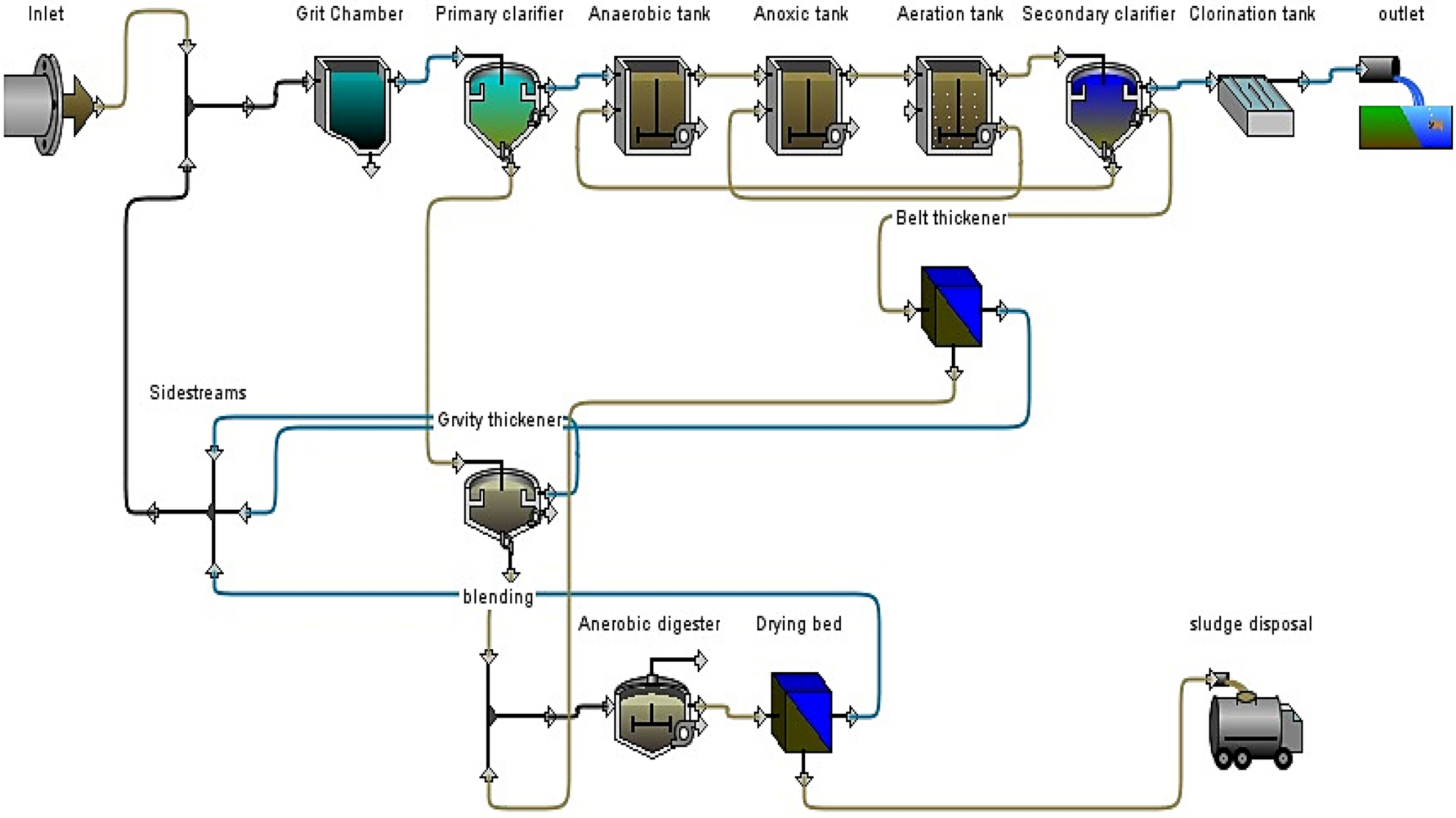The image depicts a detailed, colored diagram illustrating a multistep chemical or water refinement process on a white background. Starting at the upper left corner, the pipeline begins at an inlet and flows right, following a series of arrows that guide through each processing stage. The first stage is the grit chamber, represented by a rectangular basin. From the grit chamber, the flow proceeds into a circular primary clarifier. 

The diagram then shows the flow continuing through several interconnected tanks: the anaerobic tank, the anoxic tank, and the aeration tank. Notably, a looping pathway is indicated from the aeration tank back to the anoxic tank. Following the aeration tank, the process advances to the secondary clarifier, which has two possible directions for the effluent. One pathway leads to the chlorination tank and then exits the system as the final outlet, suggested by a downward arrow releasing water.

The alternative pathway from the secondary clarifier diverts downwards into a belt thickener and then further to the left into the gravity thickener. From here, the substance is blended and directed down towards two subsequent stages: the anaerobic digester and the drying bed, represented by another blue and black cube. Finally, the last stage involves transferring the processed sludge to a sludge disposal vehicle, completing the entire refinement sequence.